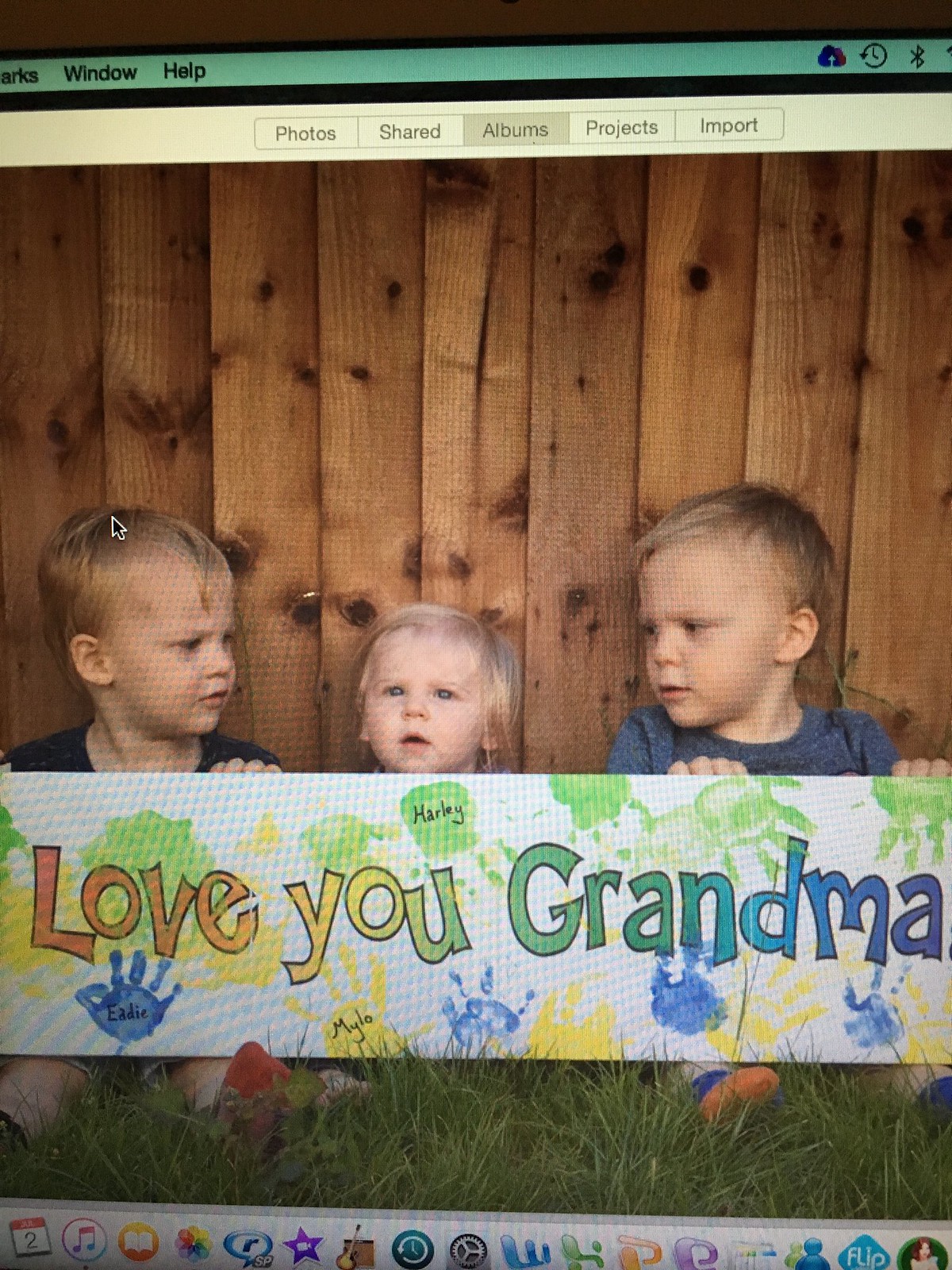This detailed image depicts a screenshot of a photo displayed on an Apple computer monitor, with visible menu options at the top reading "Window," "Help," "Photos," "Shared," "Albums," and "Import." The taskbar at the bottom also shows various icons. The photograph features three young children—two girls and one boy—sitting on grass in front of a medium-tone brown wooden fence. The children, all of whom have blonde hair, are arranged from left to right with the oldest on the right and the youngest in the middle. The child on the left has short, light-colored hair and is wearing a dark shirt. The middle child, presumably the youngest, with visible blonde hair, has an obscured shirt. The boy on the right, the presumed oldest, wears a blue shirt.

The children are holding a colorful, hand-crafted sign with the words "Love you, Grandma." The sign features a white background adorned with handprints in green, yellow, and blue. Each handprint has a name written on it: "Eddie" on the blue, "Mila" on the yellow, and "Harley" on the green. The message "Love you, Grandma" is written in a vibrant, rainbow-colored design, making it a heartfelt, personalized gift.